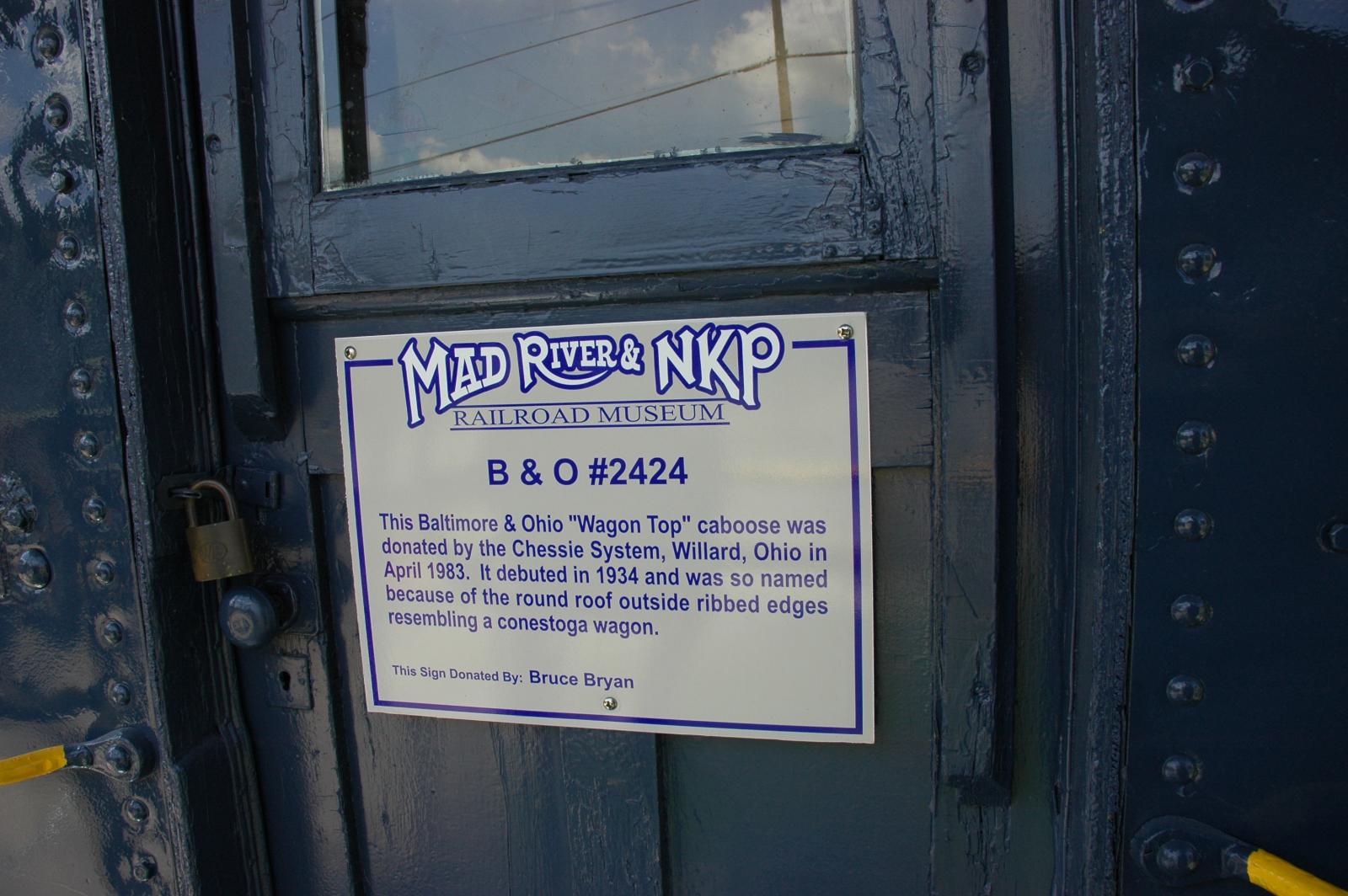This image captures a close-up view of an old, navy blue door that is centrally featured and locked with a bronze padlock. The door, which is part of the Mad River and NKP Railroad Museum, has a window at the top reflecting the sky and clouds. Below the window, in the door's center, is a metal sign screwed into place. The sign reads: "Mad River and NKP Railroad Museum, B&O number 2424. This Baltimore and Ohio wagon top caboose was donated by the Chessie System, Willard, Ohio in April 1983. It debuted in 1934 and was named for its round roof and outside ribbed edges resembling a Conestoga wagon." The sign, donated by Bruce Bryan, adds historical context about the caboose. Flanking the door are walls with rows of large rivets and metal plates, enhancing the door's rugged and historic appearance. The doorknob and keyhole beneath it are visible but are overshadowed by the more modern padlock securing the door. The colors in the image range from various shades of blue, tarnished gold, white, light gray, and a touch of yellow, all contributing to the weathered, historic look of the scene, likely captured casually by a visitor to the museum.